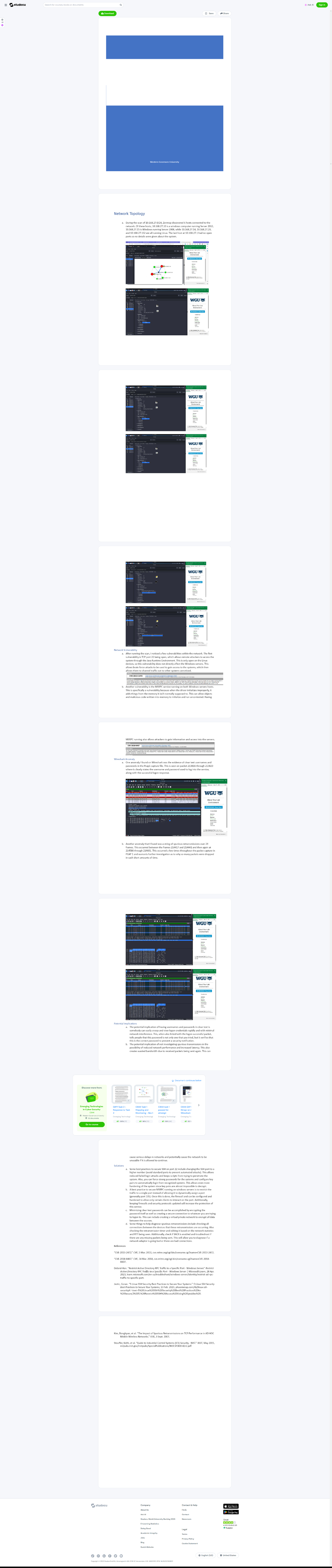This screenshot captures an elongated, narrow webpage with a densely packed layout, making individual words difficult to discern. The topmost part of the page features a thin blue line, followed by a wider white line, and then an even wider blue line. Below this, there's a gap leading to five distinct rows of black boxes. 

The first row contains two adjacent black boxes separated by a thin white line. The upper black box houses a partially opened small white box within it, and towards the right end, there's a white segment featuring blue text. The lower black box is a solid bar, with its right side containing a section topped by a blue line and accompanied by blue text. 

Following another white space, two long rectangular black boxes are situated, divided by a central white line. On the right side of these rectangles, are two white boxes; the top one is capped with a blue line, followed by another blue line below it, and a lower section with a white background and blue writing.

The complex layering of colors, lines, and boxes makes the page appear intricate and highly formatted, indicative of a structured data presentation or a formatted layout such as a spreadsheet or database interface.